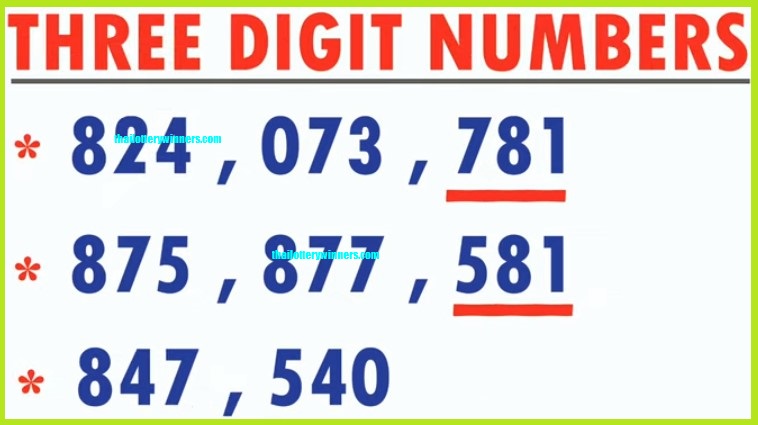The image features a sign with a neon green border and a white background, titled "THREE-DIGIT NUMBERS" at the top in red, capital letters. A red line runs beneath the title, separating it from the main content. The content consists of three red bullet points, each listing a series of blue numbers. The first bullet point includes the numbers 824, 073, and 781. The second bullet point lists 875, 877, and 581, while the third bullet point shows 847 and 540. Both the numbers 781 and 581 are underlined in red. Additionally, there are two light blue watermarks featuring website addresses, one in the center and another in the top left, though they are too small to decipher. The layout leaves space for potential additional numbers at the bottom.